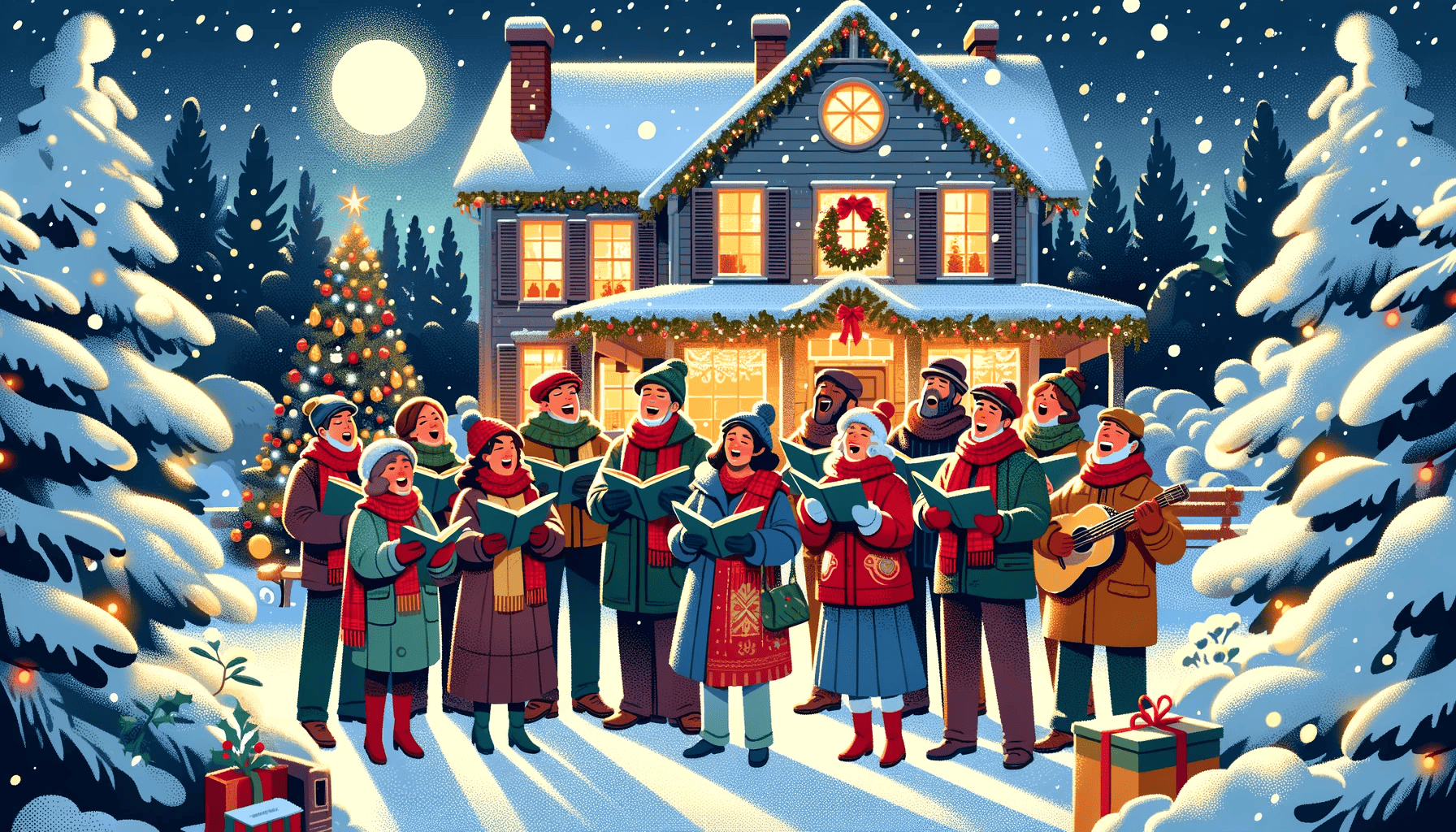This illustration, evocative of an old-timey magazine, captures a joyous group of carolers in a vibrant winter wonderland at Christmastime. The scene is richly colorful, featuring 13 carolers warmly dressed in scarves, heavy coats, boots, and hats, with the reds and greens of Christmas echoed throughout their attire and the decorations. They hold identical songbooks, and one gentleman strums a guitar. The background showcases a beautifully lit and decorated Victorian-style house with a wreath on a second-floor window and Christmas lights trimming the roof. Snow-covered trees adorned with lights and ornaments, including a large tree with a star on top and gifts under its branches, enhance the festive atmosphere. The full moon and twinkling stars illuminate the snowy night, completing this enchanting holiday scene.